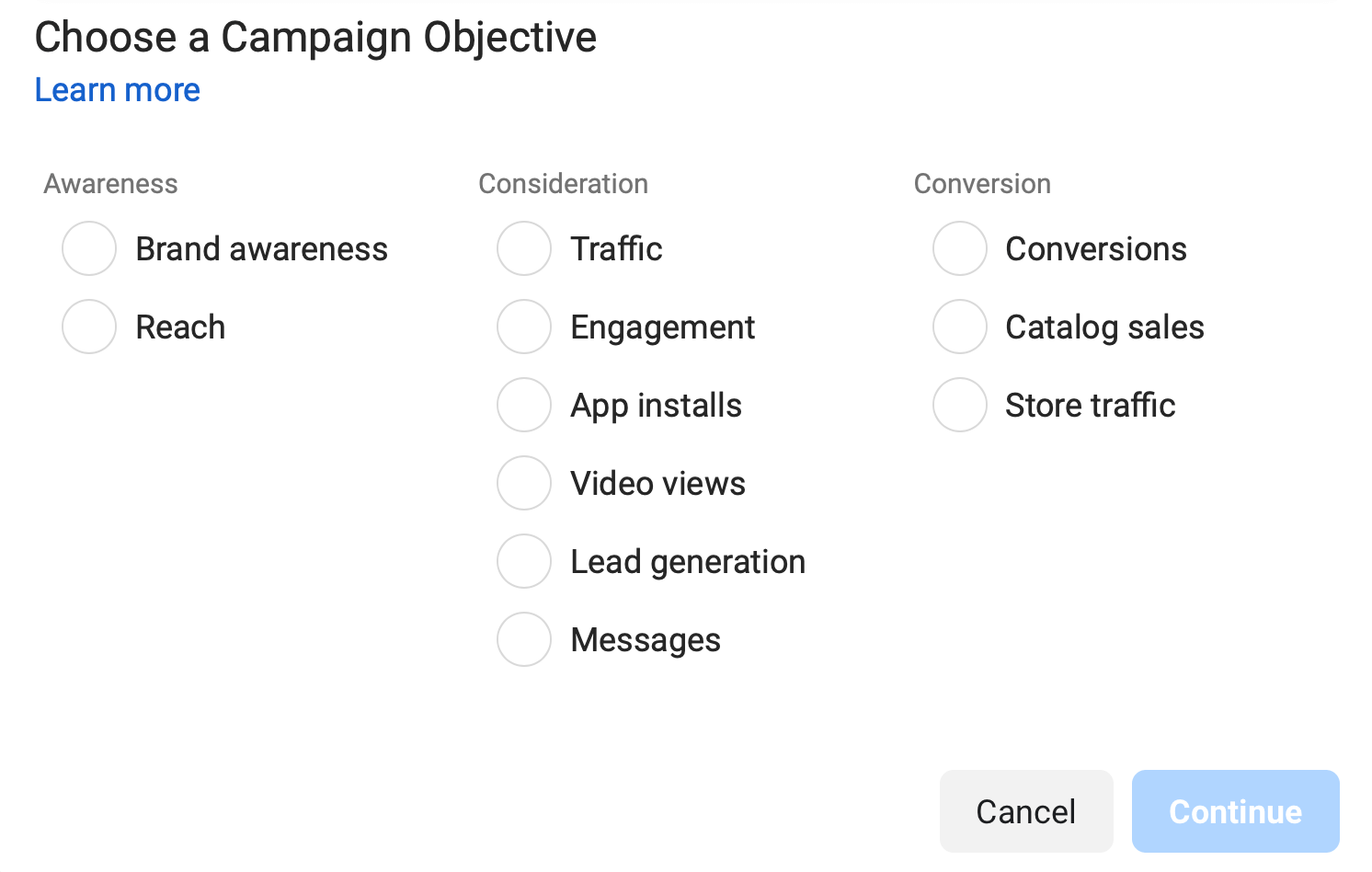The image displays a website interface focused on selecting a campaign objective. At the top, a thin gray line outlines the top of the webpage, which prominently features the title “Choose a campaign objective.” 

Below this title, a blue, clickable "Learn More" link is clearly visible. The interface is divided into three distinct categories: Awareness, Consideration, and Conversion.

1. **Awareness**:
   - **Brand Awareness**: An unselected circle next to it.
   - **Reach**: An unselected circle next to it.

2. **Consideration**:
   - **Traffic**: An unselected circle next to it.
   - **Engagement**: An unselected circle next to it.
   - **App Installs**: An unselected circle next to it.
   - **Video Views**: An unselected circle next to it.
   - **Lead Generation**: An unselected circle next to it.
   - **Messages**: An unselected circle next to it.

3. **Conversion**:
   - **Conversions**: An unselected circle next to it.
   - **Catalog Sales**: An unselected circle next to it.
   - **Store Traffic**: An unselected circle next to it.

At the bottom of the website, there are two buttons: a gray "Cancel" button and a blue "Continue" button. The "Continue" button is depicted in a muted blue color, giving it a less prominent appearance.